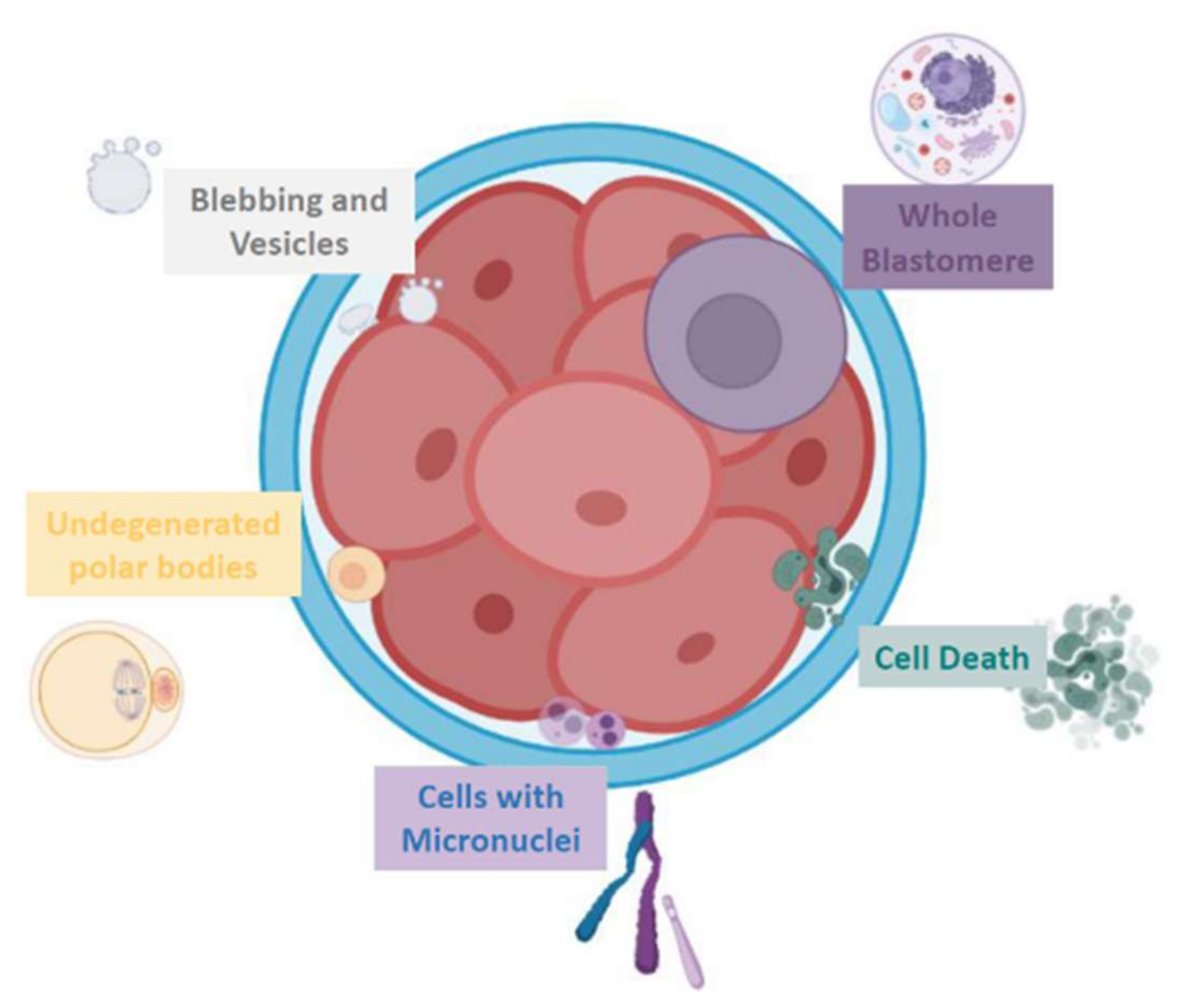The image appears to be an intricate scientific diagram, possibly from a biology textbook or science magazine, depicting various cellular structures and processes within what seems to be a petri dish. The primary feature is a large blue circle containing multiple red and dark reddish round shapes with maroon-colored ovals at their centers, suggestive of different cell types or cellular components.

In the center, there's a prominent blue area labeled "whole blastomere," surrounded by various labeled sections illustrating specific cellular phenomena. At the top left, light blue circles marked "blebbing and vesicles" can be observed. To the right, within the same blue-bordered area, the label "whole blastomere" is repeated. At the bottom right, a section titled "cell death" illustrates cells turning a greenish hue, indicative of disintegration. The bottom left corner is labeled "cells with micronuclei," highlighting small purple circles, while the left side features "undegenerated polar bodies," represented as orange circles with a darker orange center.